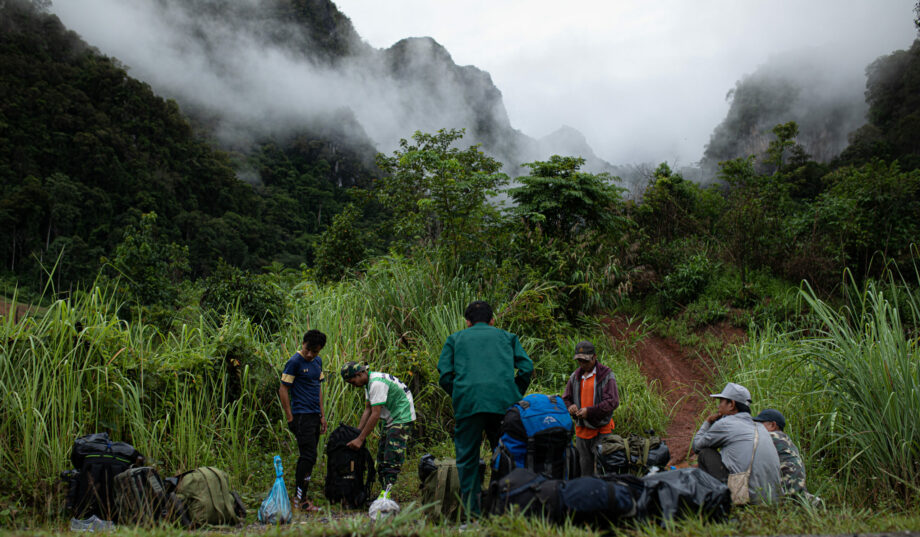In the foreground of this photograph, a group of six men is gathered, some sitting on or standing near numerous bags that are scattered around them. The men, who appear to be medium to dark-skinned and dressed in modern casual clothes, are positioned at the base of a steep incline. The setting does not resemble typical American landscapes, suggesting it might be in Asia or South America. The area is lush with six-foot-tall pale green grasses, and a red dirt path curves up the incline to the left. Behind the men is a strikingly overgrown landscape featuring enormous, steep mountains thick with vegetation. The mountainous backdrop is shrouded in mist and steam, creating a smoky, ethereal atmosphere. Dark green jungle foliage blankets the lower elevations, transitioning into a foggy upper half. A road made of dark red dirt weaves up the hills, accentuating the dense greenery and sporadically placed trees, including a prominent emergent canopy layer. This intricate blend of towering misty mountains, towering grass, and diverse greenery paints a vivid and detailed image of the scene.